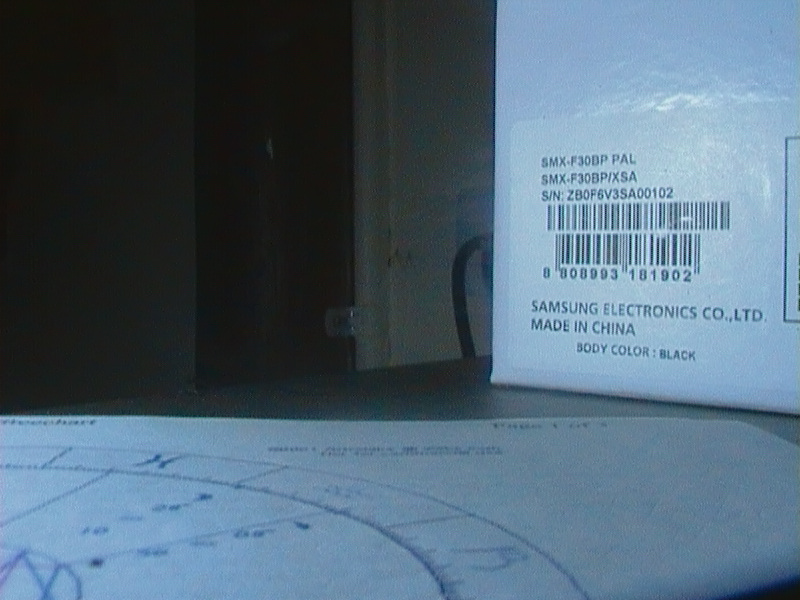The image shows a desk in what seems to be a dorm room. At the center of the desk is a worksheet or piece of paper with blue markings, likely related to navigation or measuring angles. Nearby, there's a white box prominently labeled "Samsung Electronics Co., Ltd.," made in China with the body color listed as black. This box, which could be for a TV or another electronic device, also features barcodes and various codes. The background reveals a closed door, adjacent to a white wall, and a pipe running along it. The overall scene is slightly cluttered, but the emphasis is on the desk items, particularly the worksheet and the box.